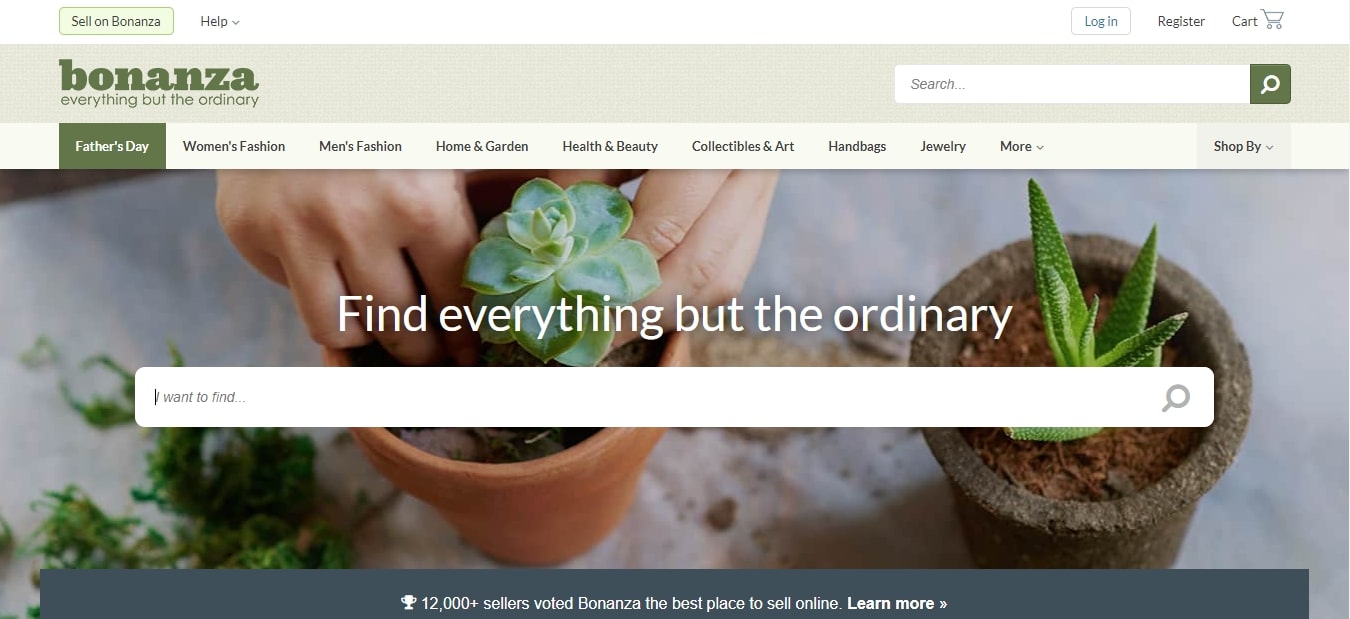The website for Bonanza features a design that combines practicality with an inviting aesthetic. At the top, a shaded grey banner stretches from left to right, featuring the branding elements. On the left side in small, dark green letters, it reads "Bonanza," with the tagline "Everything but the Ordinary" displayed just below.

Above this main banner, on the left, there's a smaller shaded panel that says "Sell on Bonanza," followed by "Help" to the right. Further along the top right, options for "Log In," "Register," and a cart icon labeled "Cart" are visible. Just beneath these options, a search bar is found under another shaded banner, allowing users to easily search for items.

Below this search bar, several categories such as "Father's Day," "Women's Fashion," "Men's Fashion," "Home and Garden," "Health and Beauty," "Collectibles and Art," "Handbags," "Jewelry," and "More" are listed. Each category is highlighted with a dark green background, except "Father's Day," which stands out with white lettering on a dark green shaded banner. Further to the right, dropdown menus for "Shop" and "Buy" with downward-pointing arrows offer more browsing options.

The main section of the page prominently features an image of a Caucasian individual planting a cactus-like plant in a brown clay planter. This scene is set against a white sheet, with visible soil and additional plants scattered around. To the right of the individual, another planter, resembling brown stone and also containing a cactus, contrasts against the white background. A central banner bisects the image with the phrase "Find Everything But The Ordinary," accompanied by a search bar prompt that reads "I want to find."

Finally, at the bottom of the image, a dark grey shaded banner claims, "12,000+ sellers voted Bonanza the best place to sell online," followed by a "Learn more" call to action.